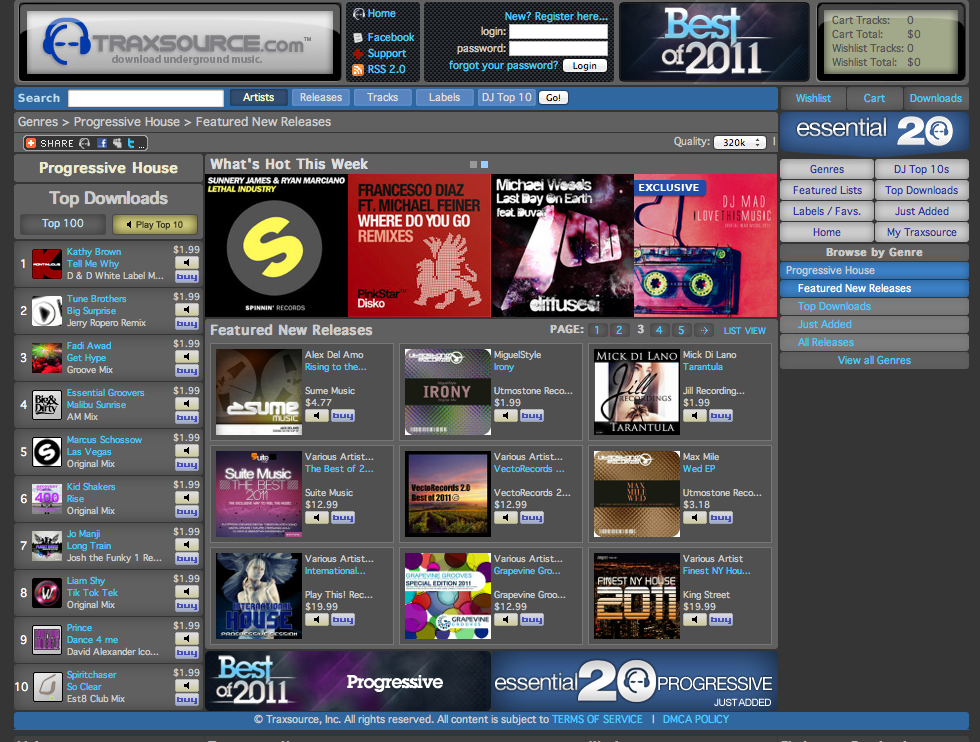The image is a detailed screenshot of the homepage of Tracksource.com, a website dedicated to downloading underground music. The top header prominently displays the website's name, "tracksource.com," alongside the tagline "download underground music." Adjacent to this, there are options for user interaction and navigation, including buttons for "Facebook support," "RSS 2.0," and user login fields for existing members and a registration link for new users.

A notable banner labeled "Best of 2011" spans across the page, highlighting the year's top music selections. Below this, there's a shopping cart section with details such as "cart tracks," "cart total," "wish list tracks," and "wish list total," providing a seamless shopping experience.

On the left side of the image, a list showcases the "Top Downloads," with ten highlighted tracks each priced at $1.99. Centrally located on the page is a prominent section titled "What's Hot This Week," featuring nine new releases arranged in a 3x3 grid format.

Additional sections labeled "Progressive Essential 20" and "Progressive Just Added" further categorize the music offerings, enhancing user navigation. The page is abundant with links, categories, and descriptive tags, ensuring that users can easily discover new and popular underground music.